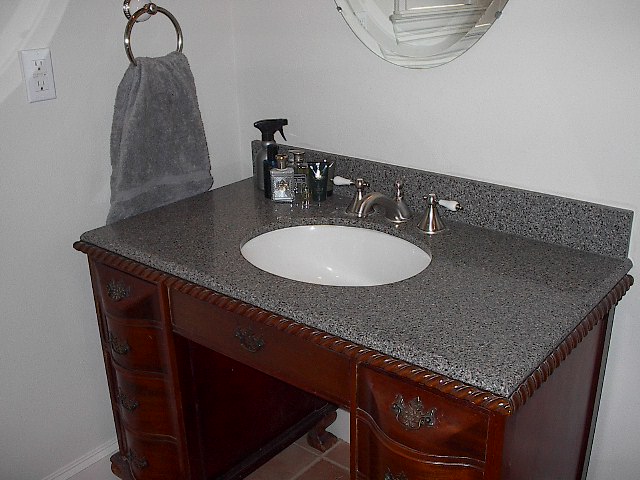The image showcases a vintage-inspired bathroom sink against a pristine white wall. At the center, partially visible, is a rounded mirror with its lower section captured in the frame. Beside the mirror, a white electric outlet and a silver towel ring holding a dark grey, fluffy towel can be seen. 

The sink itself is set within an elegantly crafted vanity that resembles an old-fashioned desk. The countertop is made of polished black granite, complemented by silver knobs with white handles that resemble miniature trophies.

A collection of men's grooming products, including aftershave, cologne, a grey spray bottle, and other toiletries, is neatly arranged on the countertop. The vanity unit is made of rich dark cherry wood, featuring ornate legs and intricate details. The central area of the vanity consists of a single door, flanked by four smaller drawers on each side. The overall setup exudes a blend of classic charm and modern functionality.